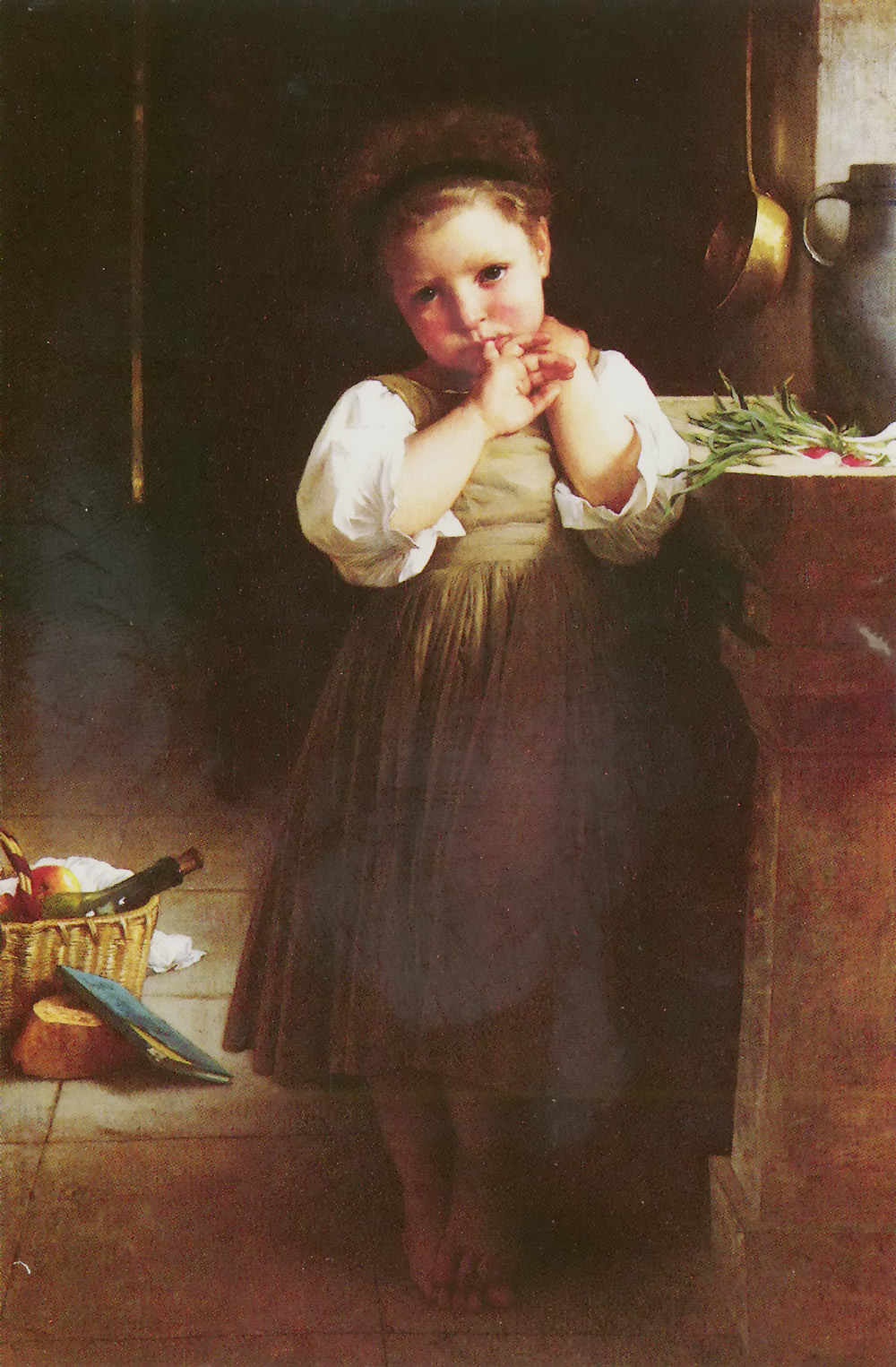The image titled "The Little Sulk" or "Little Sulky" by William Adolphe Bouguereau, created in 1871, is an oil painting in portrait orientation. It depicts a young girl, approximately four to five years old, standing in a kitchen setting. She is facing the viewer with a sad or guilty expression, her head tilted slightly to the right. Her brown hair is pulled up under a dark-colored headband or bonnet. She is wearing a long, greenish-golden dress with white puffy sleeves and a pale green apron over it. Her pinky finger is in her mouth, and her left hand is placed behind her neck. She is barefoot, with her feet crossed at the bottom of the image.

The background features various kitchen elements: to the right, there is a straw basket containing food items, including a bottle of wine with a cork, and possibly a fruit or apple, along with a white cloth. To the left, on a counter, lie green onions or herbs, and a gray vase. A copper skillet hangs on the wall behind the vase. The overall scene is illuminated against a dark background, highlighting the details of the girl's attire and the kitchen setting. The style of the painting is vintage portraiture.